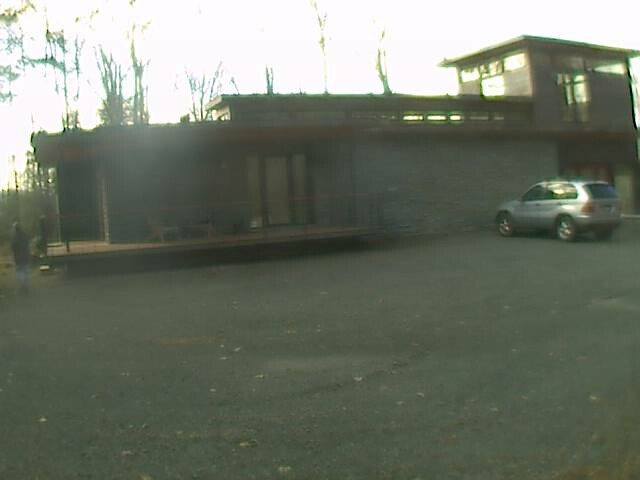The photograph depicts the exterior of a uniquely designed, square-shaped house with a blend of wooden and brick construction. The house features a wooden deck with two chairs on the left side, a glass and brick paneled tower for a second floor, and a half-floor storage area extending to the left. Central to the structure is a section of concrete and on the right are striking red double doors. Light filters down at an angle, illuminating the scene without revealing the sky.

In front of the house, there's an asphalt driveway or parking lot where a silver SUV, possibly a late-2000s to early-2010s model, is parked. On the left side of the building is a person wearing dark blue clothing and blue jeans, though details are blurry. The background is dotted with thin, spindly trees, likely palm trees, adding a touch of greenery to the scene. The overall feel of the architecture resembles something inspired by Frank Lloyd Wright, blending modernist elements with a unique personal twist.